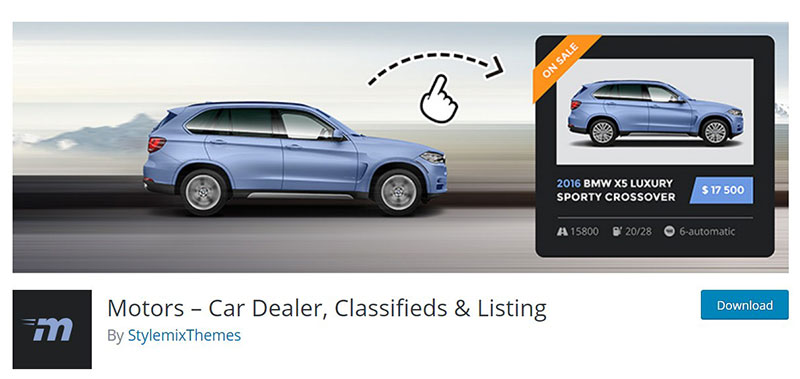The image depicts a section of a car dealership website or app interface. Dominating the top portion of the image is a prominent photograph of a blue 2016 BMW X5, a luxury sporty crossover SUV. Accompanying this image is a detailed information box to the right, stating the car's price of $17,500 and its mileage of 15,800 miles. Fuel efficiency information is also provided, indicating a range of 20 out of 28 MPG. The car is noted to have a six-speed automatic transmission. At the bottom-right corner of the screen, there’s a section labeled "Motors - Car Dealer Classifieds and Listings," with additional options to "Buy, Style, Mix, Themes." Beside this text is a prominent blue download button, suggesting the availability of a corresponding app. An eye-catching arrow with a pointing hand icon is also present, directing attention to another image of the same car marked "On Sale."